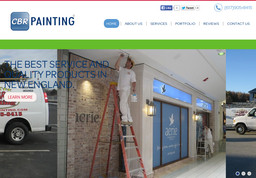The image depicts the homepage of a business website for CBR Painting. At the very top, a thin red line is followed by the text "CBR Painting" in white and blue. Directly beneath the red line, icons for Facebook, Twitter, a blue phone icon, and a contact number appear, though the number is too blurry to read.

Below this, a navigation menu in blue lists several tabs including "Home," "Contact Us," and "Reviews," among others that are hard to discern. Further down, a green line appears under which there is a slogan written in navy blue, stating "The Best Service and Real Products in New England," though part of this text overlaps with an outdoor photograph, making it partially obscured.

The main section of the image features a photograph divided into two parts. On the left side, there is a red and white box with the text "Learn More," showing a partial view of a van, a parking lot, and a blue sky. On the right side, a man dressed in a white shirt and pants stands on an orange ladder, painting the underside of a building. A doorway to the business is also visible, flanked by white columns. Additionally, there are two white circles and a blue circle suggesting another parking lot view. The font used on the website is somewhat difficult to read.